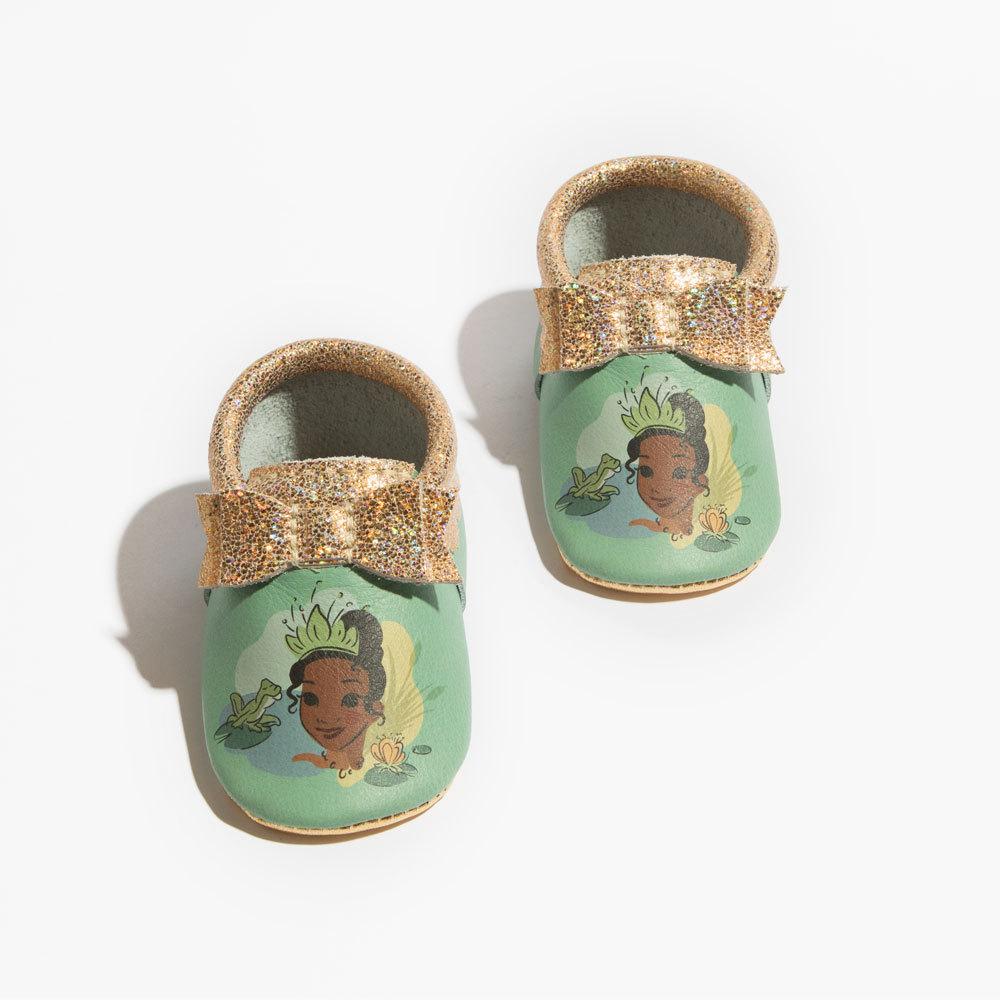The image displays a pair of infant shoes, primarily designed for young babies. These delicate shoes feature a soft sole and are predominantly pale green with a glittery gold accent trim. At the front, there are matching gold bows made from the same fabric as the trim. Notably, the shoes are adorned with a simplified, 2D animated illustration of Princess Tiana from Disney's "The Princess and the Frog." Princess Tiana, depicted in a loose line art and cell shading style, wears a green tiara and smiles gently at the frog prince, who puckers his lips toward her. Additionally, a butterfly is perched on a lily pad beside the characters, adding to the whimsical scene. Behind the illustration, there is a subtle background featuring light green, grayish, and orange hues, along with faint outlines of pond brush, enhancing the enchanting theme of the design. The shoes are photographed against a white background with a light source casting soft shadows around them.